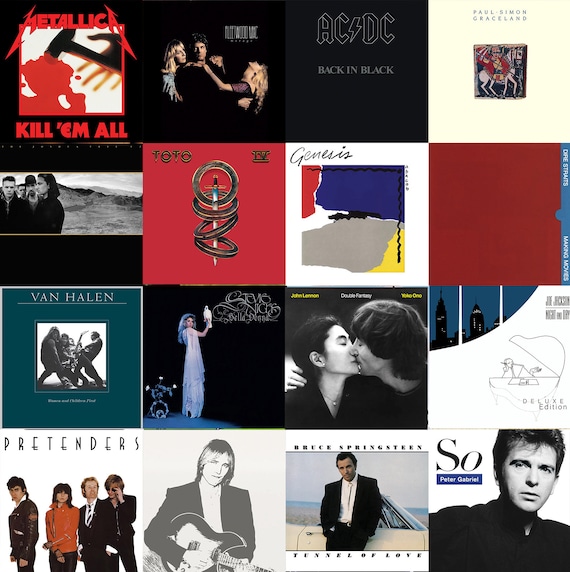The image features a meticulously arranged 4x4 grid of iconic album covers from the 70s and 80s, showcasing a variety of influential artists and bands. Starting from the top left, we see Metallica’s "Kill 'Em All" with its distinct black background and red lettering. Next to it is an album with an image of a man flanked by two women. Following that is ACDC's "Back in Black," characterized by its stark, minimalist design, and then Paul Simon's "Graceland," which features a medieval-style sketch of a man on a horse. 

The second row begins with an album featuring a black and white photo of three men in the center, although the title is unreadable. Adjacent to it is Toto's "Toto IV," followed by Genesis’s self-titled album, and an album with a maroon cover and a horizontal teal line with white text, likely Dire Straits' "Making Movies."

In the third row, we recognize Van Halen's album cover followed by Stevie Nicks' "Bella Donna," depicted with her holding a bird while dressed in a flowing gown. Next is John Lennon and Yoko Ono's "Double Fantasy," showing the couple kissing, and Joe Jackson's album, notable for its drawn piano image with "Deluxe Edition" in the text.

The bottom row showcases The Pretenders' self-titled album with its simple white background, followed by an image in black and white of a man holding a guitar, which is Tom Petty. Next is Bruce Springsteen's "Tunnel of Love," slightly blurred but identifiable, and finally, Peter Gabriel's "So," featuring a clear portrait of the artist against a white background.